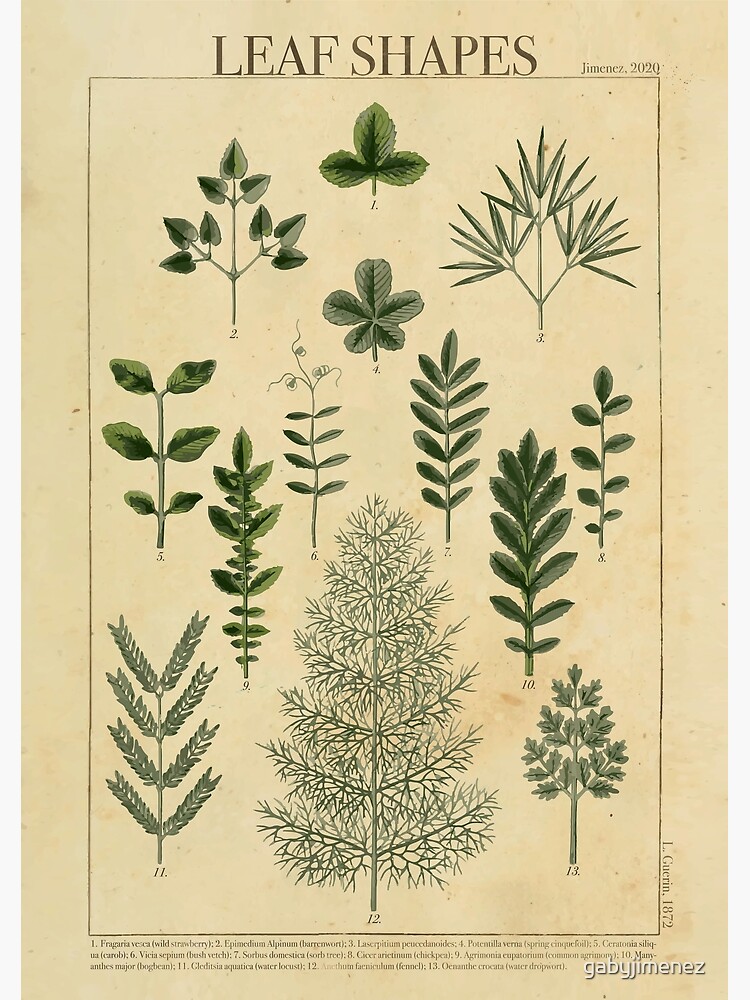This detailed caption accompanies an intricately designed poster by the artist Gabby Jimenez, titled "Leaf Shapes." The poster, characterized by its faded beige tone accented with deliberate wear markings, evokes a sense of timelessness. Centered within a rectangular inset that leaves ample borders on all sides, the poster features an array of diverse leaf shapes meticulously illustrated. Prominently centered within this collection is a full branching tree, notably devoid of leaves, which adds an intriguing focal point to the composition. The top of the poster is adorned with the title "Leaf Shapes," while a smaller inscription at the bottom reads "Jimenez 2020," providing the creator's name and the year of creation. The entire artwork, rendered with a vintage aesthetic, invites viewers to appreciate the elegant simplicity and variety of natural forms.